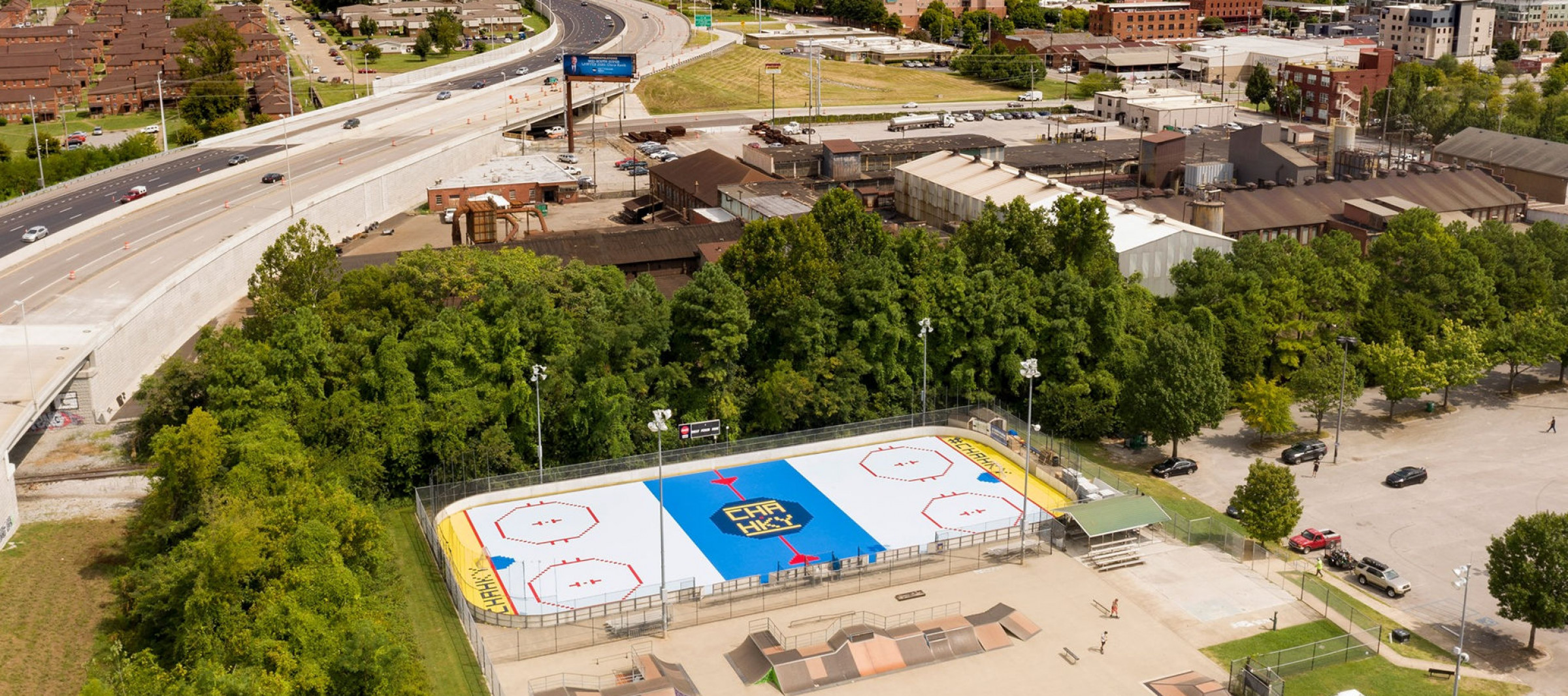This drone aerial photograph captures a cityscape highlighting multiple key features. On the left side of the image, a newly paved black highway with concrete barriers and sparse traffic runs adjacent to a housing complex featuring identical cookie-cutter houses with brick fronts and chocolate brown roofs. To the right, a secondary road connects to the highway and is lined with cars. This road stretches past another housing complex with white fronts and gray roofs, both complexes bordered by dark green trees.

Prominently centered in the image is a walled-off rink area, most likely for roller hockey, marked with yellow text reading "CHA HKY" with red arrows through it. The rink is adorned with red hexagonal shapes at the top and bottom, and triangular dark blue shapes within yellow rectangles. Further right, there is a skate park with two figures, amidst a parking lot and people walking near tents. 

Beyond these recreational areas, two industrial parks span across the landscape. The first features buildings with varied facades—brick, stone, and concrete—while the second has largely worn-down brown structures and a substantial white building extending towards a large tree line. An industrial area with office buildings and smokestacks is visible in the background, and various cars are parked and moving through the scene. This snapshot presents a dynamic city park as its focal point, reflecting the intermingling of residential, recreational, and industrial zones. 

For more information, visit www.fema.gov.